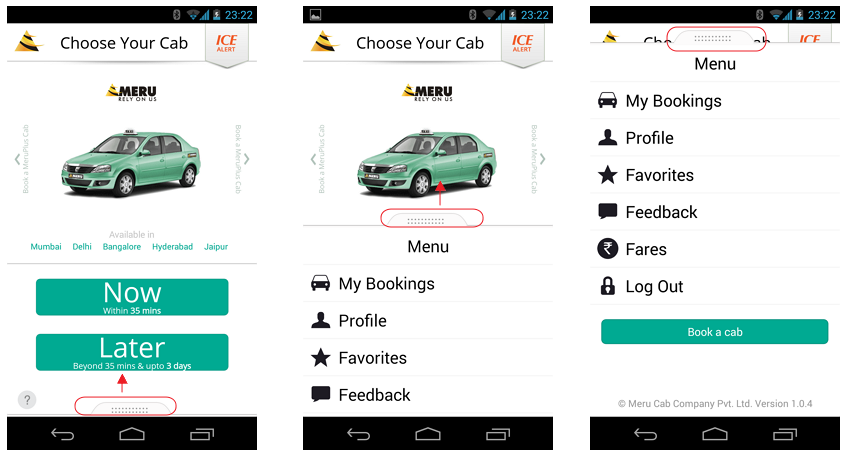The screenshot depicts a website interface showcasing three different options for booking a cab. Every option contains a consistent black tab at the top and bottom of the screen, providing essential icons for battery, Bluetooth, time (which is 23:22 on all three), Wi-Fi signal, and cellular strength.

The central portion of each option features a white background with the headline "Choose your cab." The first and second options include an "Ice Alert" banner beneath this headline. The first option specifically lists "Meru" as the cab service, indicating its availability in Mumbai, Delhi, Bangalore, Hyderabad, and Jaipur. Below this, there is a banner that informs users of the service's booking windows: "Now within 35 minutes," "Later beyond 35 minutes," and "Up to three days," with a highlighted red circle and an upward-pointing arrow emphasizing the "Later" option.

The second option also displays a red circle with an upward-pointing arrow, but here it directs attention to a car icon. There is a drop-down menu labeled "Menu," which includes the following options: "My Bookings," "Profile," "Favorites," and "Feedback."

In the third option, the "Choose your cab" headline is partially concealed by an expanded drop-down menu. This menu includes "My Bookings," "Profile," "Favorites," "Feedback," "Fares," and "Logout." Additionally, beneath the menu, there is a button prominently displayed against a green background with white text that reads "Book a cab."

Overall, the image provides a detailed comparison of the cab booking options available on the website, highlighting specific features and menu options within each segment.